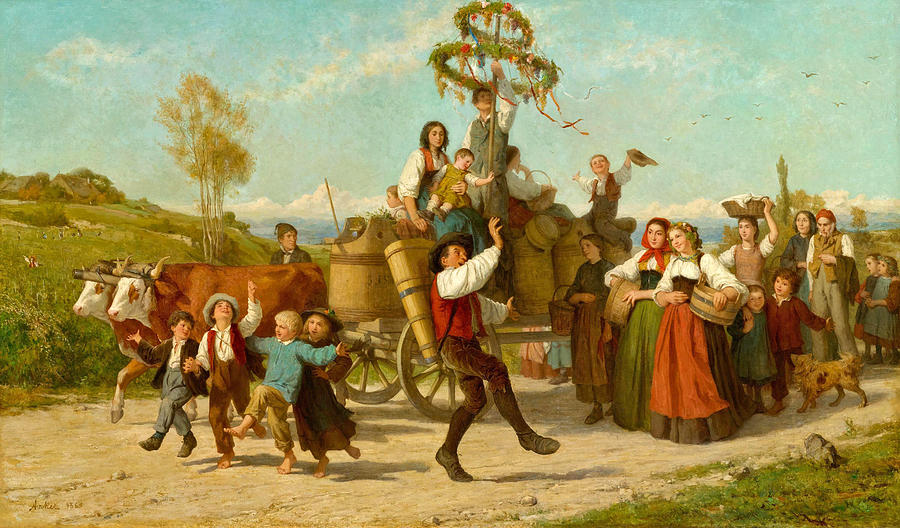The artwork is a detailed painting capturing an outdoor celebration scene, set under a clear blue sky with a few fluffy clouds. It features a lively crowd of people, all dressed in traditional attire; the women are in long skirts with bustiers and white shirts, while the men sport vests, white shirts, pantaloons, brown leather trousers, and boots. Central to the image is a road on the left side, where a man in a black hat and red vest is loading items onto a wagon pulled by two oxen. The wagon, carrying large wooden barrels and various cargo, has children, a woman, and a man sitting on top. The man on the wagon holds a pole adorned with wreaths and ribbons fluttering in the wind. In the foreground near the wagon, children are playing and dancing, accompanied by a man dancing behind them. The left side of the scene also features fields of grass, trees, and a house, while the bottom right includes grassy and rocky areas. Two brown and white cows can be seen in the background near the road. The artist's signature, possibly "anchor," is located in the bottom left-hand corner.